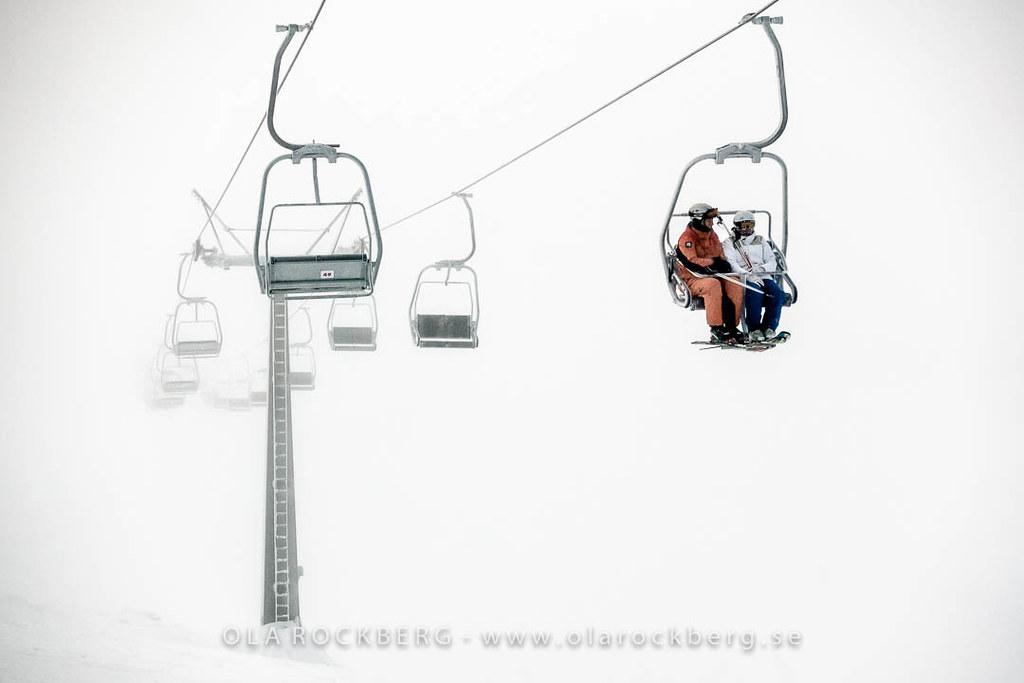The image captures a ski resort tram system with the trams riding on high wires amidst a snowy, white background. Most of the trams are empty, except for one tram in the front right which has two people on it. One person is dressed in an orange and black ski outfit, while the other is wearing a white helmet, a white puffy jacket, and blue pants. Both have skis on their feet with ski poles resting in their laps. The tram system has two sides, with trams moving in opposite directions, and as the tram line extends into the distance, the scene becomes misty, suggesting fog on the mountain. This atmospheric detail adds a layer of intrigue to the overall scene. At the bottom of the image, a watermark reads "Ola Rockberg - www.olarockberg.se".